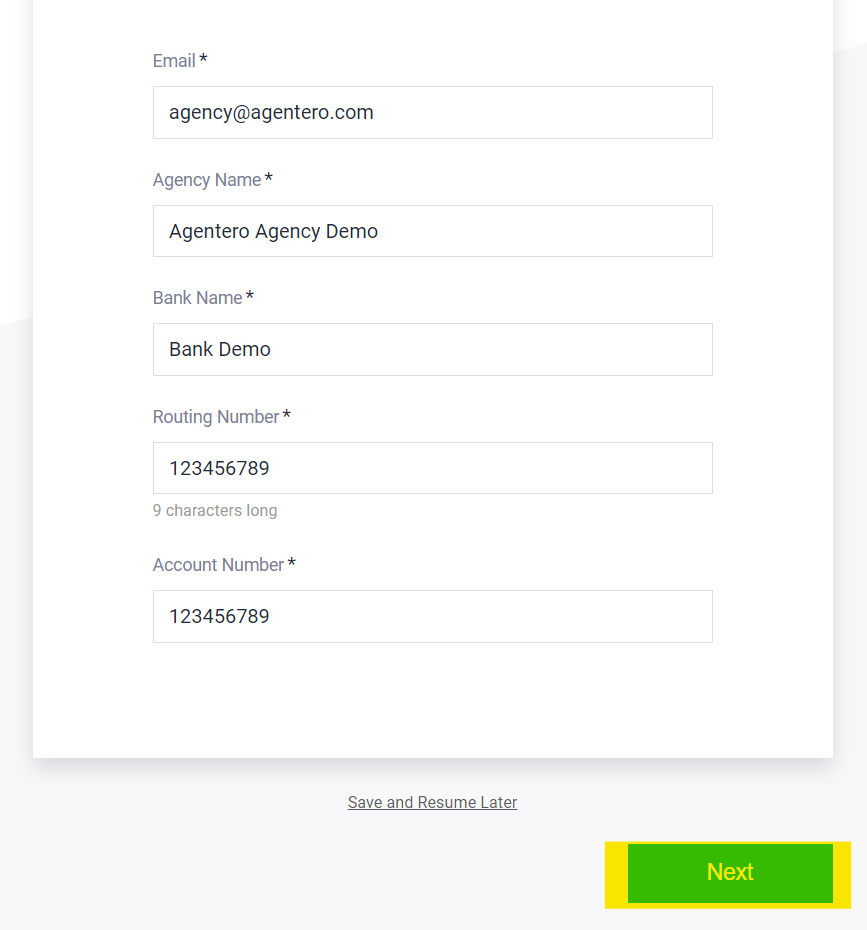In the image, the central focus is a form featuring five key categories, each neatly arranged from top to bottom. The categories, initially presented in a subtle gray text, include 'Email', 'Agency Name', 'Bank Name', 'Routing Number', and 'Account Number'. Corresponding entries are displayed in bold black text, providing specific information: the 'Email' field is filled with "agency@agentero.com", under 'Agency Name' it reads "Agentero Agency Demo", in the 'Bank Name' category, the text says "Bank Demo", and both the 'Routing Number' and 'Account Number' fields contain the sequence "123456789".

Each category and its respective information are encompassed within long, thin rectangles adorned with a delicate gray outline. These rectangular fields are uniformly positioned one below the other, creating a structured and organized layout. The entire form is framed by a light gray border that neatly encapsulates all the elements, providing a sense of completion and focus. The image itself rests upon a pristine white background, enhancing the clarity and readability of the text.